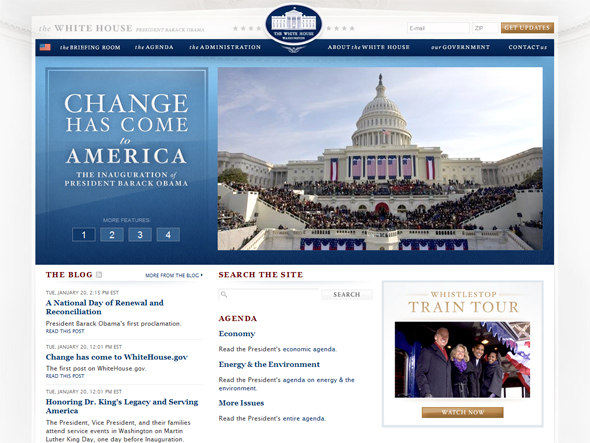Screenshot of a webpage from the White House website, capturing a detailed and organized layout:

- The header prominently displays "The White House" followed by a series of varied images.
- Central image features the U.S. Capitol adorned with numerous American flags, with a large audience gathered for the inauguration of President Barack Obama. Overlaid text reads, "Change has come to America, the inauguration of President Barack Obama."
- Below, a "More Features" button is displayed with selectable numbers 1 through 4.
- A "Blog" section is visible, showcasing headlines in blue text.
- On the right side, a "Search the Site" option includes an input box for searching.
- An "Agenda" section outlines key topics with linked descriptions in blue text:
  - "Economy: Read the President's economic agenda"
  - "Energy and the Environment: Read the President's agenda on energy and the environment"
  - "More Issues: Read the President's entire agenda"
- A dedicated page for the Whistle Stop Train Tour, complete with a gold "Watch Now" button.
- At the bottom, there is a field to enter an email and zip code to receive updates.
- Design elements include a blue banner and a predominantly white background interspersed with blue and occasional red text.